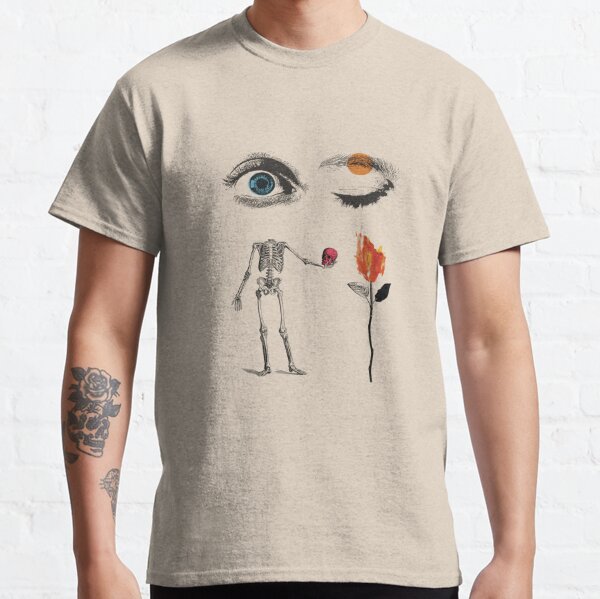This image features a torso-only view of a man, as it is cropped just below his neck, so his head and face are not visible. He is wearing a light brown-beige t-shirt, revealing his neck and arms down to his wrists. His pants are partially visible at the top and appear to be black. His hands are positioned off-screen and not visible.

The t-shirt has a distinctive and detailed design. On the left side of the shirt, there is an open eye with a blue eyeball. Directly below this eye, a headless skeleton is depicted. The skeleton, rendered in black and white etching, is holding a pink skull in its outstretched left hand. In contrast, the right side of the t-shirt features a closed eye. Below the closed eye, there is an illustration resembling a flower with a flame-like appearance in shades of orange and yellow. Above this closed eye is a yellow circle that looks like either the sun or the moon.

The man has noticeable tattoos on his right arm, with designs including a skull and a rose, primarily in dark blue to black ink. The tattoos cover significant portions of his arm, enhancing the detailed aesthetic of his appearance in the image.